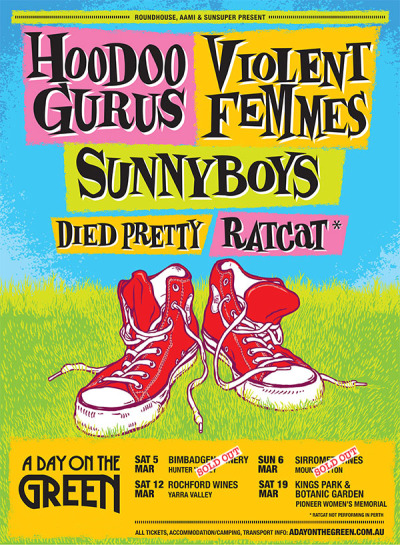The colorful animated poster features a vibrant blue sky as the background, symbolizing an animated scene, with lush green grass along the lower half. Prominently displayed in the foreground are untied, red high-top Converse Chuck Taylor shoes resting on the grass. The poster announces a series of concerts with bold black text outlined in white, dividing band names and event details against various colored backgrounds. At the top left, the featured bands include Hoodoo Gurus against a pink backdrop and Violent Femmes on the right with a yellow backdrop. Below these, the band names Sunny Boys appear with a yellow background, followed by Died Pretty on the left and Rat Cat on the right. At the bottom of the poster, within a yellow box, the event details are listed: "A Day on the Green." Dates and venues mentioned include Saturday, March 5th (sold out), Sunday, March 6th (sold out), Saturday, March 12th at Rochford Wines in Yarra Valley, and Saturday, March 19th at Kings Park and Botanic Garden, Pioneer Women's Memorial.